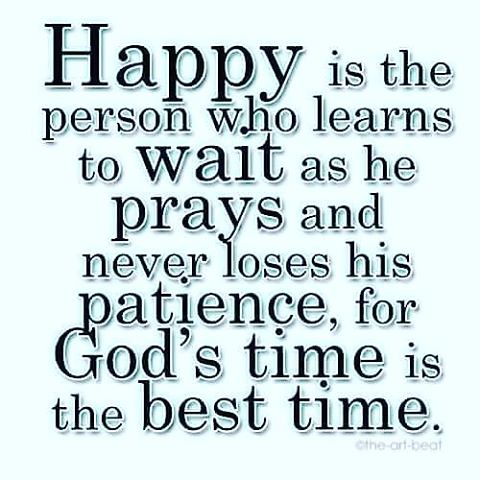This image features a religious phrase centered on a simple, light blue (teal-tinted) transparent background. The phrase is written in black text with a white outline and spans eight lines. It reads: "HAPPY is the person who learns to wait as he prays and never loses his patience. For GOD'S time is the best time." The text is neatly arranged down the center of the background, and below the phrase, it is signed with "Alphart Beat." There are no other images or embellishments within the square-bordered background, emphasizing the significant and faithful message conveyed by the text.